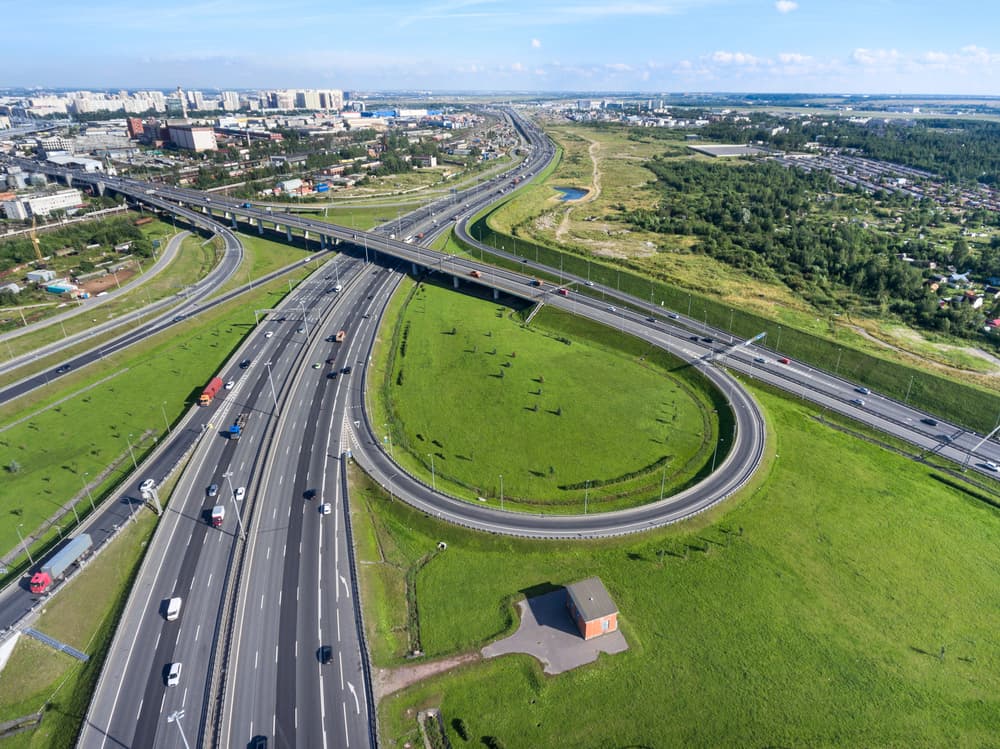This aerial shot captures a major highway that bisects the landscape, starting from the lower left and extending towards the upper horizon. The highway consists of four lanes, two heading north and two heading south. At the center of the image, a loop off-ramp curves gracefully, providing an alternate route. Below this looping ramp, nestled near the bottom center of the frame, stands what appears to be a single building, possibly a house. To the right, there's a thin river or perhaps an artificial canal that runs vertically down the image, flanked by trees and smaller residences. Dominating the upper left is the sprawling city with tall, predominantly white buildings, contrasting against the blue sky and white clouds on the horizon. The bottom left is characterized by open grassland, while the upper right features a densely wooded area with moderate development.